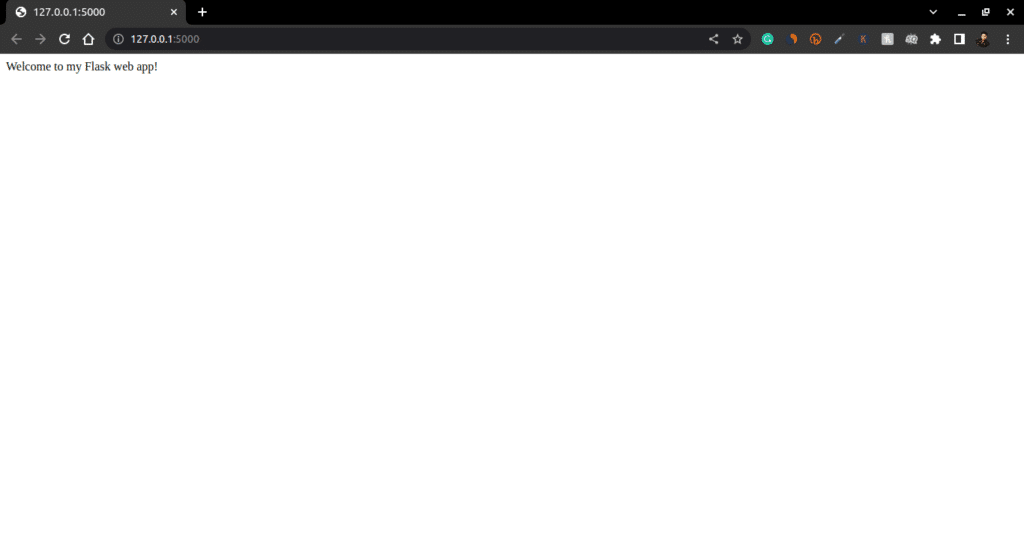The image is a screen capture of a website displayed on a web browser. The website itself is minimalistic, featuring a blank white background with a single line of black text in the upper left corner reading, "Welcome to my Flask web app!" The majority of the screen is occupied by this white space, creating a stark and uncluttered visual.

The browser's frame, which is visible as a thin bar at the top of the screen, is dark gray and black. It includes white text on the open tab, showing the URL "127.0.0.1:5000," which is also displayed in the browser's address bar. On the right side of the browser's frame, there are standard navigation items for minimizing, maximizing, and closing the window. Beneath these are several colorful buttons representing different browser extensions, including light blue, two orange, white, and gray ones.

On the left side of the browser's address bar, there are navigation icons for back, forward, refresh, and home. These icons are also white against the dark gray background of the browser frame. The simplicity of the web page, with its single line of text against an otherwise blank canvas, emphasizes the basic functionality of the Flask web application being showcased.